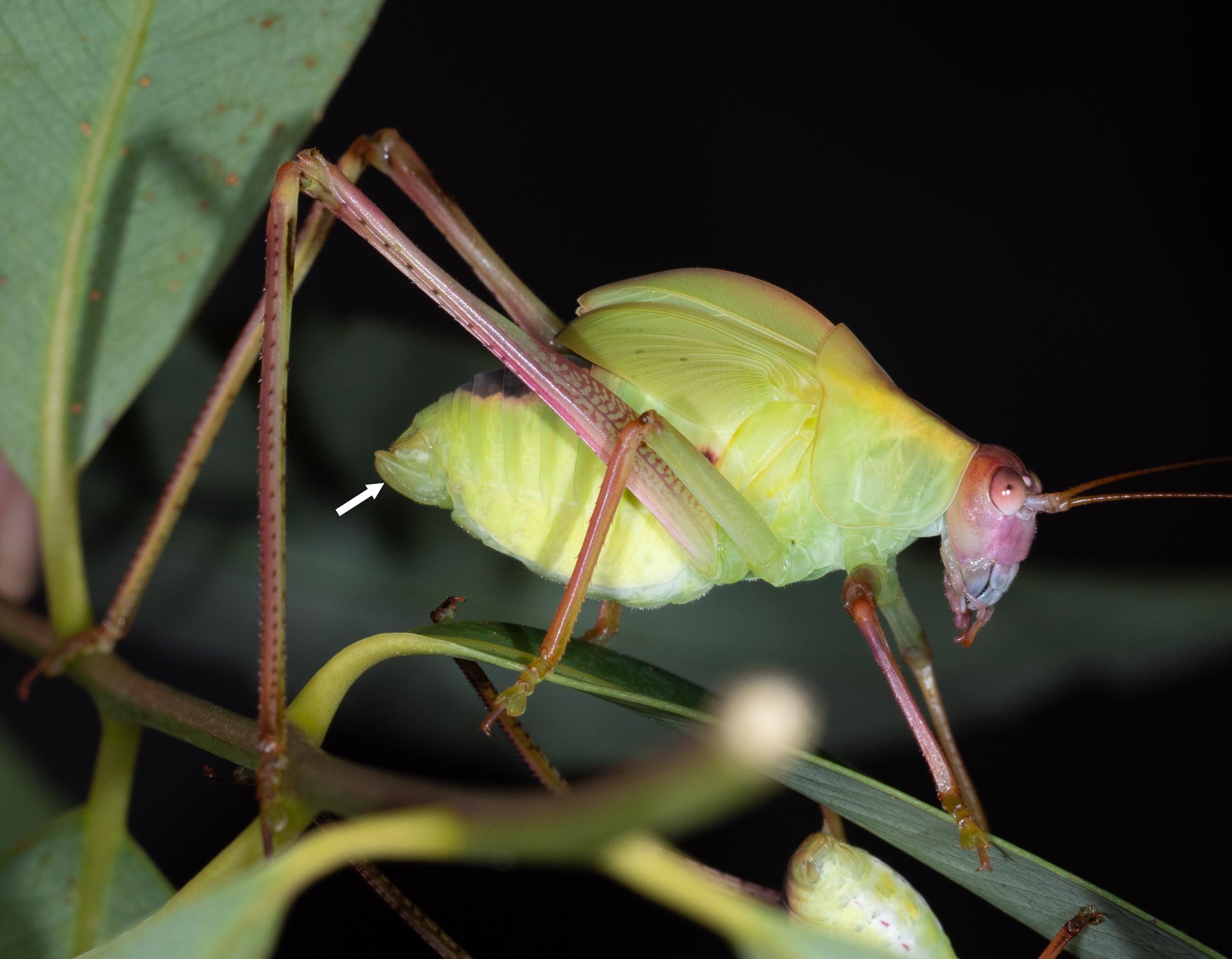The image showcases a highly detailed, side-profile shot of a small, green insect with a distinctive pinkish head and large, elongated back legs. The front four legs are noticeably shorter than the prominent back pair, which is angled backwards, highlighting the bug's unique stance as it stands on a green leaf or blade of grass. The insect, which has two thin antennae and notably pink dot-like eyes, appears to be exerting enough weight to bend the grass blade it's perched on. The head and legs exhibit a pinkish-purple hue, adding a vibrant contrast to its predominantly green body and wings. A white arrow points to the insect's rear, further emphasizing this area. The image is well-focused on the colorful, moist-looking insect, set against a blurred, blackish background with hints of leaves, twigs, and ambient nighttime lighting. There is no text, only the visual cue of the arrow. Notably, the photograph captures a moment outdoors and potentially features another similar bug on the underside of the grass.